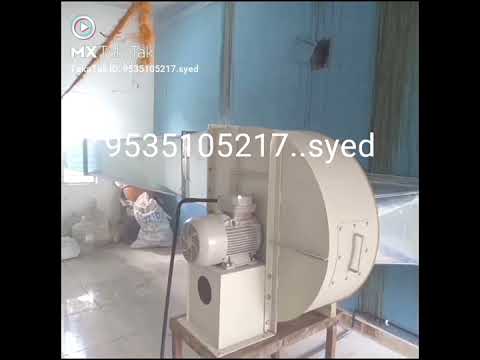The photograph depicts a large piece of industrial equipment, likely a blower or some sort of generator with a motor mounted to it. The machine, predominantly white or beige-gray in color, is situated in a room with a blue wall and a light gray, tile floor. Metal ductwork is connected to the machine, suggesting it functions as part of an HVAC system or similar setup. In the background, there's a bag and possibly a jug of water on the floor. Superimposed over the image are white text and black vertical bars framing the photo. Central to the image, the text reads "9535105217...SYED". In the upper left corner, more white text is visible but partially obscured, displaying "MX something TAC," and there is a white circle with a right-facing arrow next to it. The entire scene is characterized by its industrial setting and unclear purpose, with visual cues suggesting its function related to air or fluid movement.